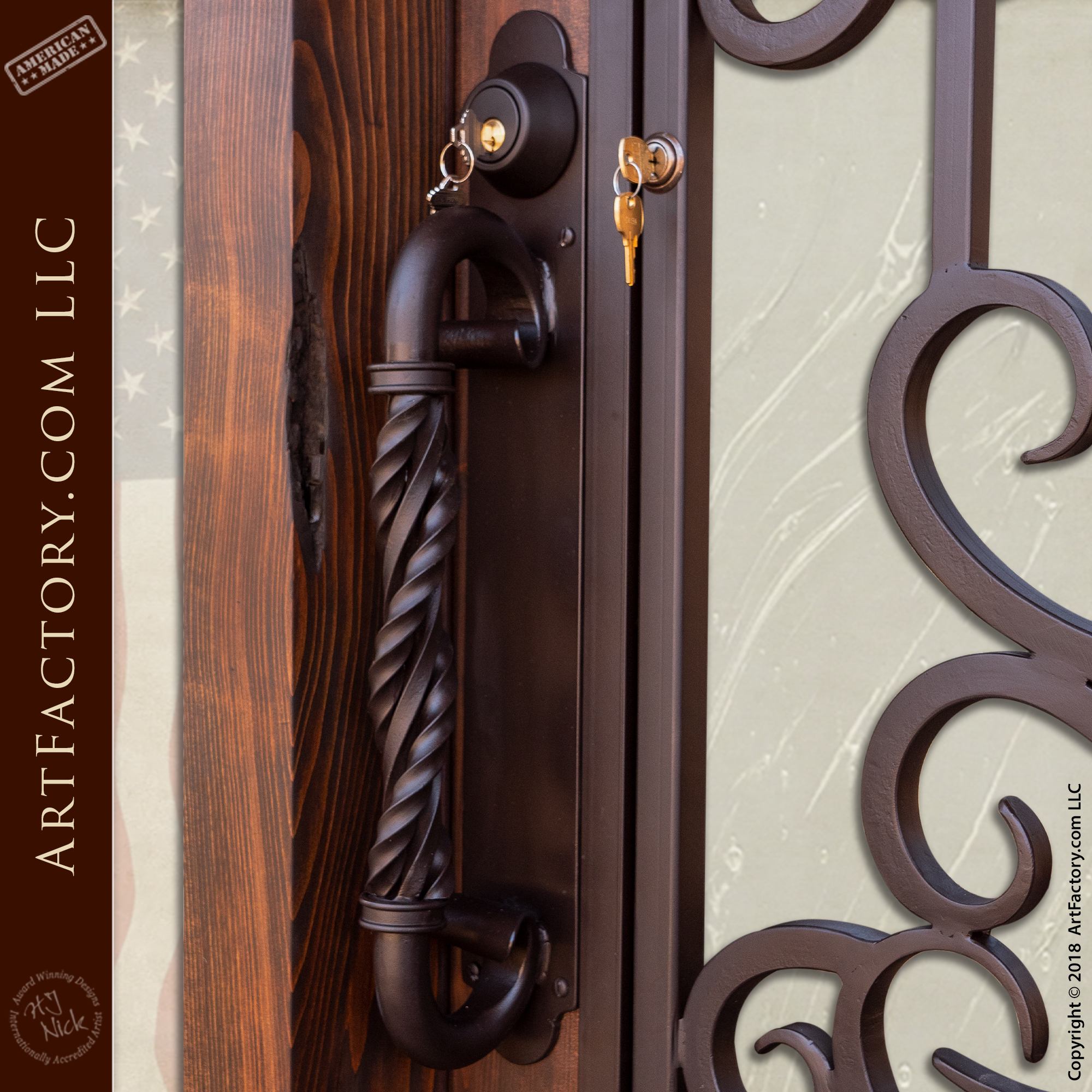This detailed photograph captures an opulent, heavy-duty front door with rich design elements that convey a sense of luxury. The door, framed by a variety of finely crafted wooden panels, features an intricate dark brown handle with an elaborate spiral pattern, reminiscent of a twisted iron rod. Above this striking handle, there is a black lock with a silver key inserted, and to the right, an additional lock is visible, also with a key inserted and a matching key hanging down. The left side of the image showcases informative text on a brown border, displaying "ArtFactory.com LLC American Made" in gold lettering. At the bottom right corner, small black letters note "copyright 2018 ArtFactory.com LLC." The overall composition highlights the craftsmanship and the elegance of the door, with special attention to the detailed metalwork of the handle and locks.